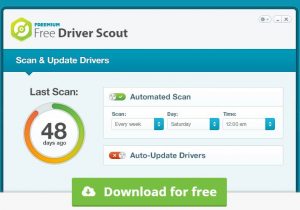The image depicts a pop-up window for a free driver update tool called "Driver Spout." The design primarily utilizes dark blue and green colors. At the top, there is an icon for the application followed by text, which is partially obscured but prominently displays "Free Driver Spout" in black lettering. 

On the far right of the window, there are menu option buttons including an "X" to close, a minus sign for minimizing, and an unreadable third button. Below these buttons is a blue bar labeled "Scan and Update Drivers." 

The interface also shows the status of the last scan, conducted 48 days ago, represented by two concentric circles—one white and another that partially fills with green and orange segments, possibly indicating progress or usage over time.

A narrow box is available for filtering options, and a toggle button indicates that "Automatic Scan" is enabled. Further down, there are three dropdown menus specifying scan intervals: set to scan every week, on Saturdays, at 12:02 a.m. Additionally, there is another toggle button for enabling "Auto Update Drivers."